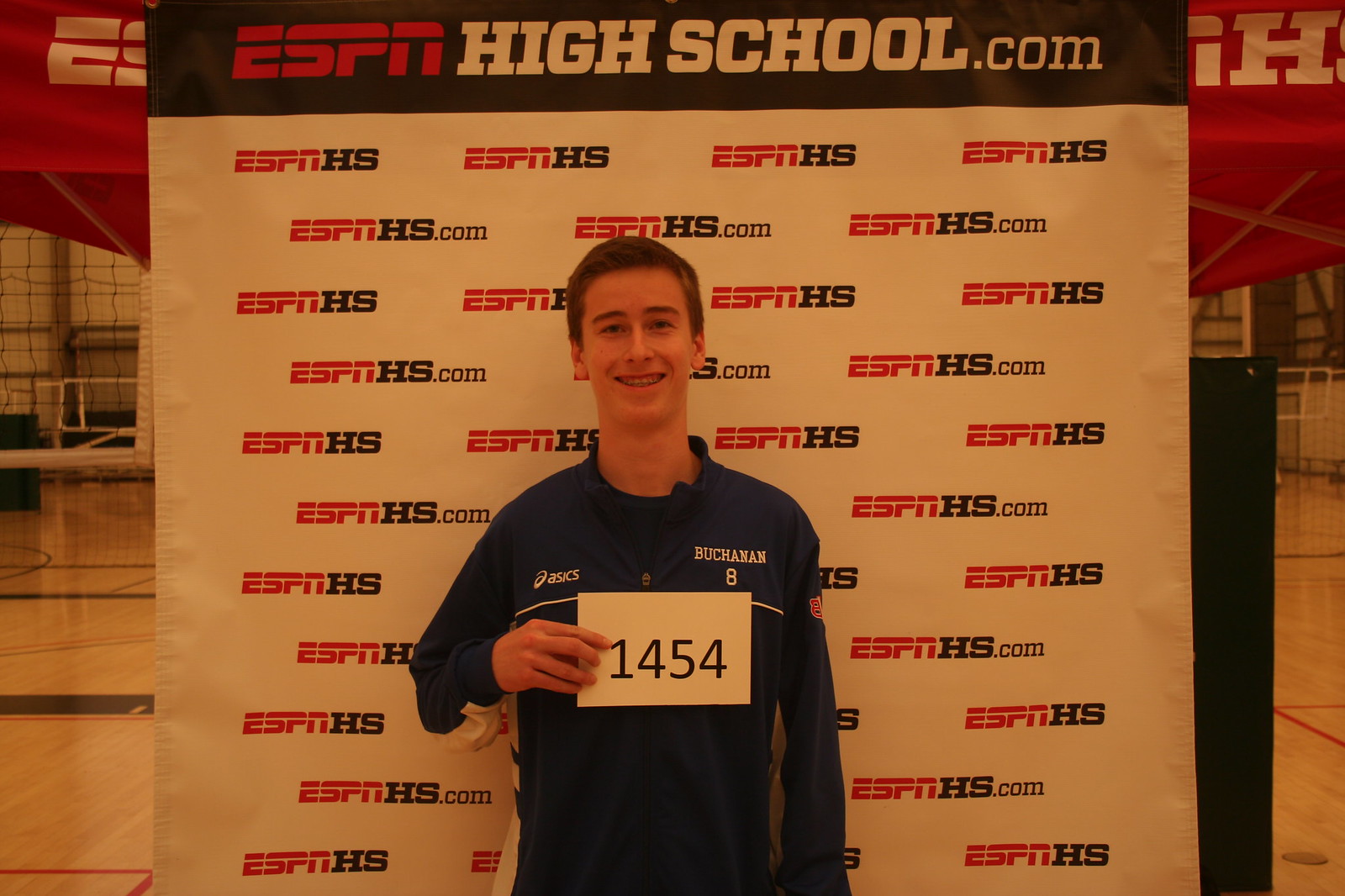In this photo, a young man, likely 17 or 18 years old, is standing in front of a gymnasium backdrop. The backdrop consists of a large, drop-down banner with a black border at the top, displaying "ESPN" in red and "highschool.com" in white. The banner's background is white and features a repeated pattern of "ESPNHS" and "ESPNHS.com" text. In the gymnasium behind him, you can see the shiny, light tan floor typically found in such settings, along with volleyball nets and a red awning tent, also marked with "ESPNHS."

The young man, who has short, light brown hair and braces, is smiling broadly. He is wearing a long-sleeve navy blue A6 brand sports jersey with his name, "Buchanan," and the number eight on it. In his right hand, he holds a white card with the number 1454 written in black.